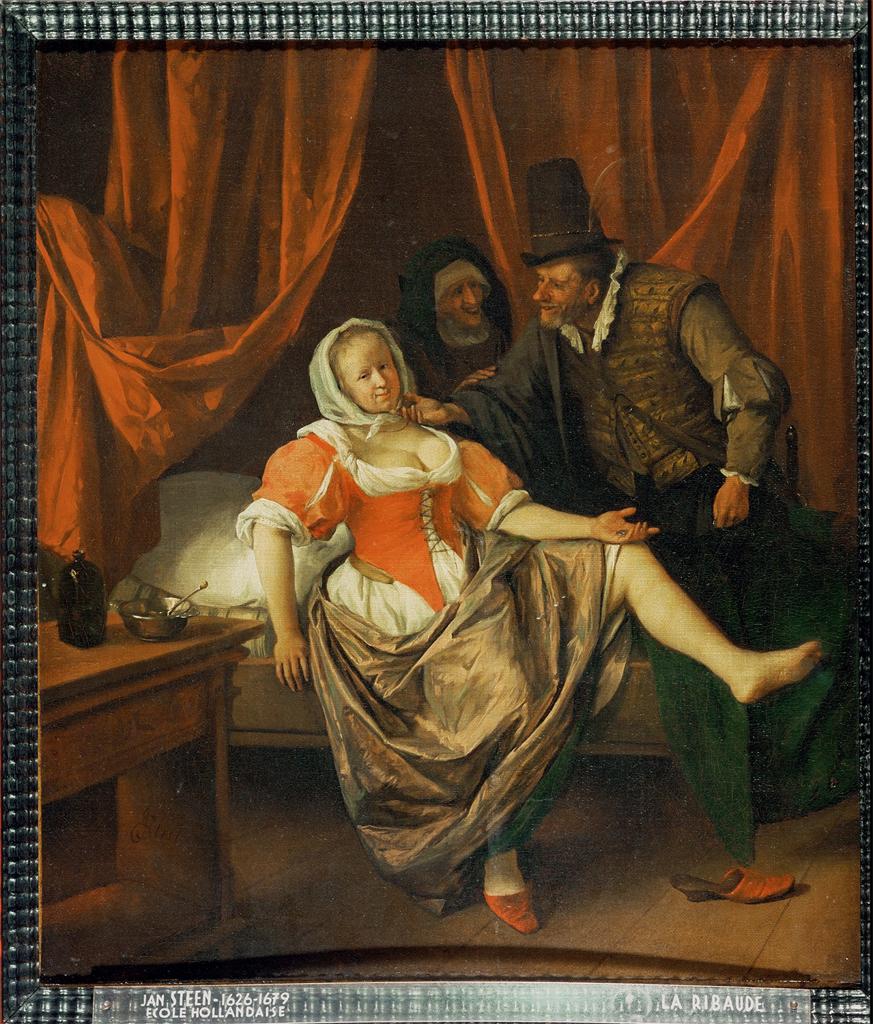This artwork, resembling an antique or Renaissance painting, depicts a scene with three figures against a backdrop of orange drapes that fall from the ceiling. Foregrounded is a woman reclining on a canopy bed, dressed in an elaborate orange and white corset over a white skirt, partially covered by a brown overskirt. She wears a white cloth hood, tied elegantly under her chin. Her right leg, adorned with a red heel, rests on the floor, while her bare left leg is propped up on the bed, revealing her skin from knee to toe. Her right arm supports her as she leans back, while her left arm rests on her raised knee. 

A man sits behind her, garbed in traditional Renaissance attire including a brown vest with puffy sleeves, a black cape, and a brown long top hat. He appears to be examining the woman, gently touching her chin. To their rear, a woman dressed as a nun, with a white cloth hood under a black veil and brown robes, observes the scene. In the foreground, there is a wooden table displaying a silver plate, a jar of medicine, and a black glass bottle with a spoon sticking out, suggesting a medicinal context to the scene. The setting is completed by a wooden floor, grounding the tableau in a period-appropriate ambiance.